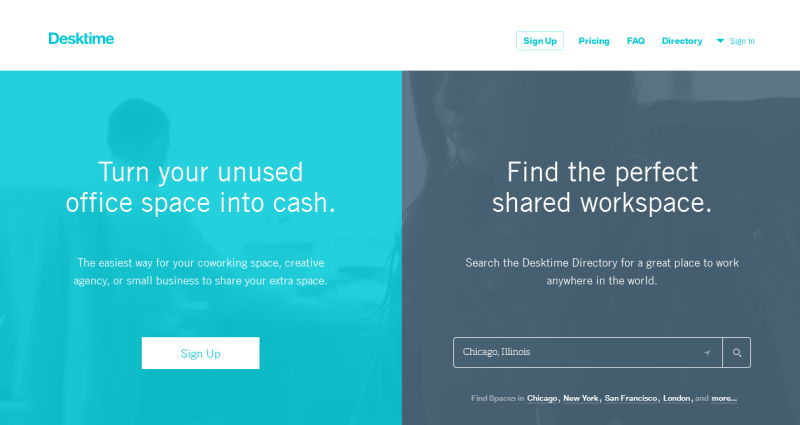This advertisement for the website Desktime features a visually engaging layout divided into two prominent colored sections. On the left side, a bright teal square displays a central white text message that reads, "Turn your unused office space into cash." Beneath it, slightly smaller text explains, "The easiest way for your co-working space, creative agency, or small business to share your extra space." At the bottom center of this teal section, a clickable white button with teal text says "Sign Up." The background subtly includes a silhouette of a person in what appears to be a typical office setting.

On the right side, a dark gray square features a central message in white text: "Find the perfect shared workspace." Below this, more detailed white text advises, "Search the Desktime directory for a great place to work anywhere in the world." Directly beneath is a search bar with "Chicago, Illinois" pre-filled, suggesting users can find spaces in cities such as Chicago, New York, San Francisco, London, and more.

The Desktime logo appears in small teal text at the top left corner on a white background. The top right corner has navigational buttons labeled "Sign Up," "Pricing," "FAQ," and "Directory" with a downward arrow indicating a dropdown menu, along with a "Sign In" option for returning users. 

Overall, the advertisement comprehensively highlights Desktime's services, guiding both potential space renters and seekers with clear, actionable prompts.